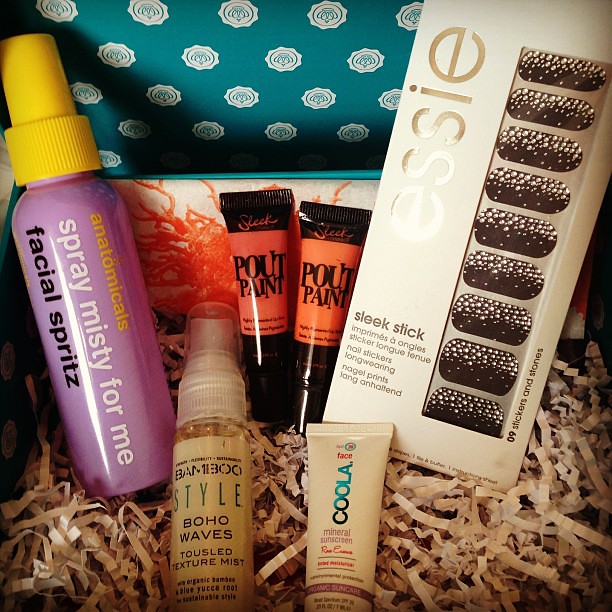This close-up color photograph depicts a curated collection of skincare and beauty products neatly arranged inside a decorative gift box. The inside lid of the box is light blue or turquoise with a pattern of small white logos resembling a crown, lending a soft, elegant backdrop to the scene. The bottom of the box is cushioned with shredded white paper strips, serving as a protective and aesthetic base for the products.

Positioned prominently on the left side, a tall pink bottle with a yellow spray top stands out. The text on the bottle, rotated 90 degrees clockwise, reads "anatomicals" in yellow, "spray misty for me" in white, and "facial spritz" in black. To the right of this bottle, two identical black tubes with orange accents, labeled "pout paint," are placed side by side.

Lying down towards the center-right of the box is a smaller clear spray bottle with yellowish-brown liquid inside. The white text on this bottle reads "bamboo style boho waves tousled texture mist." Next to it, slightly below, there is a small light brown tube bearing the brand name "COOLA" (C-O-O-L-A) in a gradient from black to light blue, labeled as mineral sunscreen. 

Finally, on the far right, leaning against the back, a tall rectangular box contains sleek stick-on nail decorations from the brand "SESIE." The box is white with black oval shapes, featuring various shiny dots. This meticulous arrangement highlights each product, making for an inviting and visually appealing presentation.